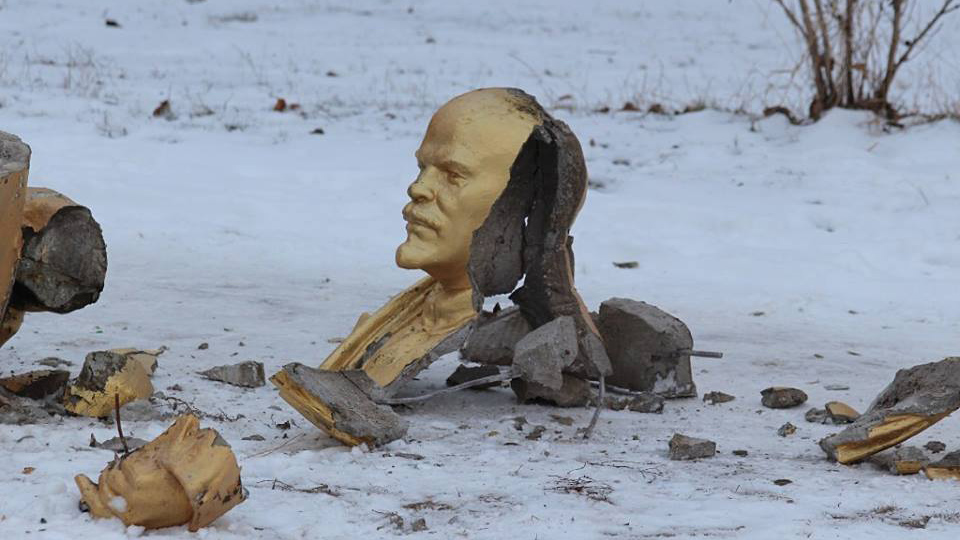In this horizontal rectangular image, a broken concrete statue lies strewn across a snow-covered ground, with a few strands of dead grass and shrubs poking through the white blanket. The statue, originally painted gold with a cream-colored exterior, portrays a man—identifiable as a bust of Joseph Stalin—with a prominent mustache. The head, broken in half, reveals a dark gray interior of cement and iron rods. Pieces of the statue, including parts of the hand, are scattered around, with chunks of concrete and rebar visibly protruding from the shattered remains. Despite the damage, the face remains largely intact, showcasing the eyes, nose, jawline, and mustache of the figure. The background features a sparsely vegetated field, with dried bushes and plants visible amidst the snow, enhancing the desolate and abandoned atmosphere of the scene.